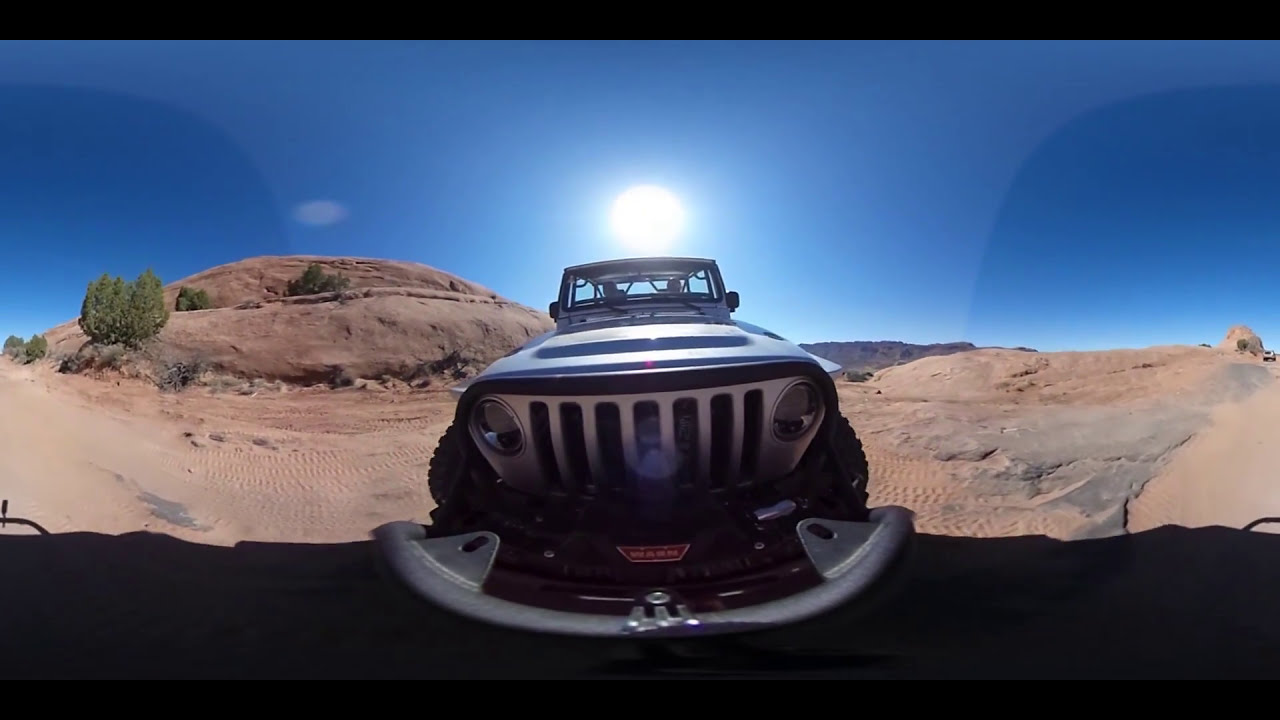This is a close-up shot of a rugged, off-road vehicle, specifically a silver-blue Jeep, prominently featuring its distinct silver grille and round headlights that resemble eyes. The elaborate front bumper is designed to facilitate attachment for towing or pulling. The Jeep's large traction tires are well-suited for the sandy terrain it is navigating. The setting is an arid desert landscape, highlighted by the presence of a cactus-like plant on the left and scattered rocks around. Behind the Jeep, a bright sun sits almost perfectly centered above the vehicle's roof against a clear, blue sky. The image, taken with a slight fisheye effect, distorts and emphasizes the silver grille against the surrounding environment. To the Jeep's left, there is a rocky hill with two levels and some green bushes, while to the right, there is a flatter, rocky area, both covered in light brown sand. Tracks left by the Jeep crisscross the sandy ground, adding to the scene's dynamic feel.